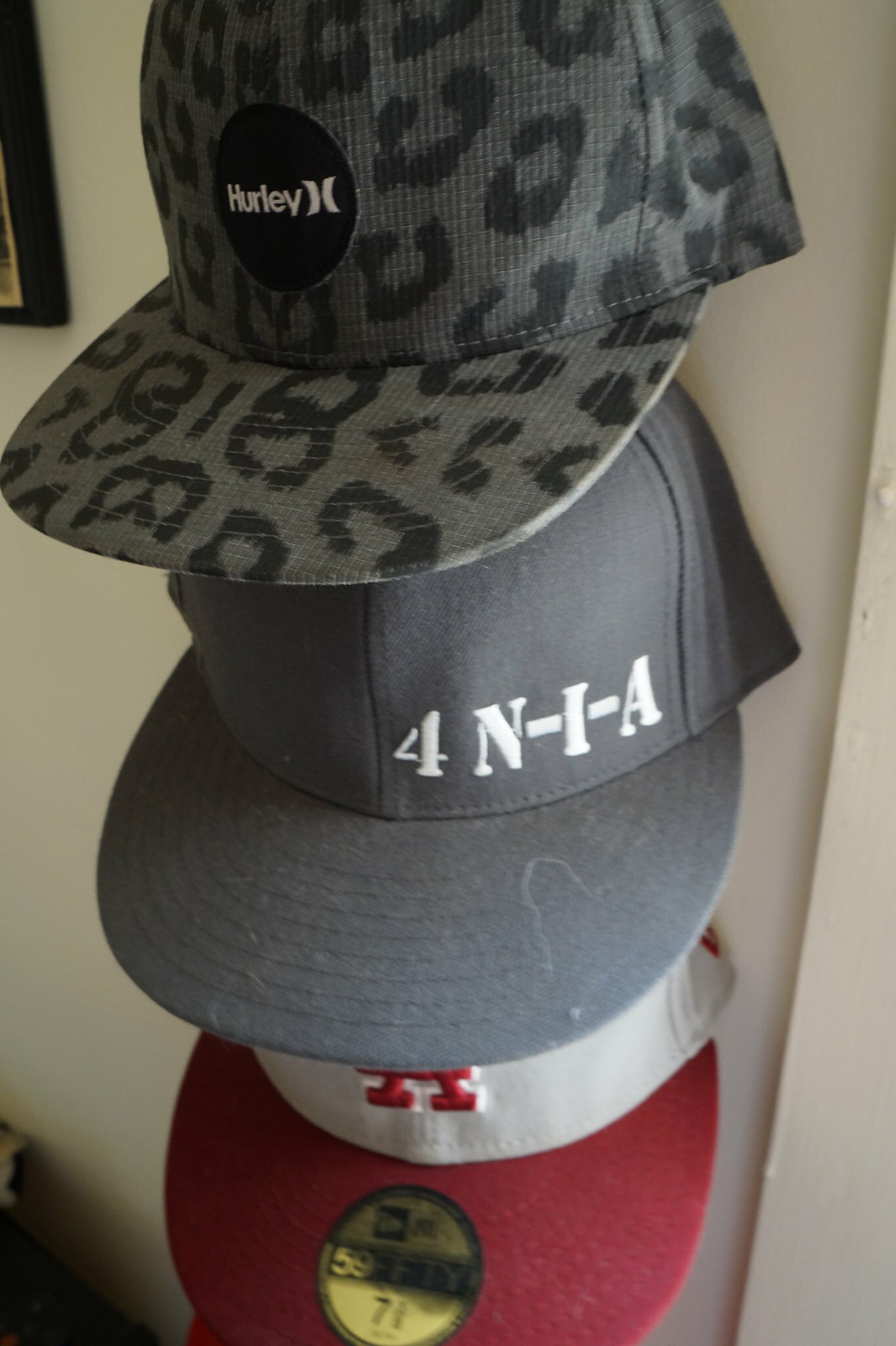This image features three baseball caps stacked on top of each other, hanging against a wall with a background that transitions from a green hue on the left side to a deep tan on the right, featuring a range of colors including brown, grey, and reddish lines. The top hat displays a grey and black leopard print pattern with "Hurley" written in white on a black circle. The middle hat is solid grey with "4NIA" stitched in white. The bottom hat has a white top with a red brim, featuring a circular emblem outlined in black with a yellow center and black stripe, indicating it's a New Era 7 1/4 size fitted hat. The overall setting appears to be indoors, with the hats decoratively mounted on the wall.